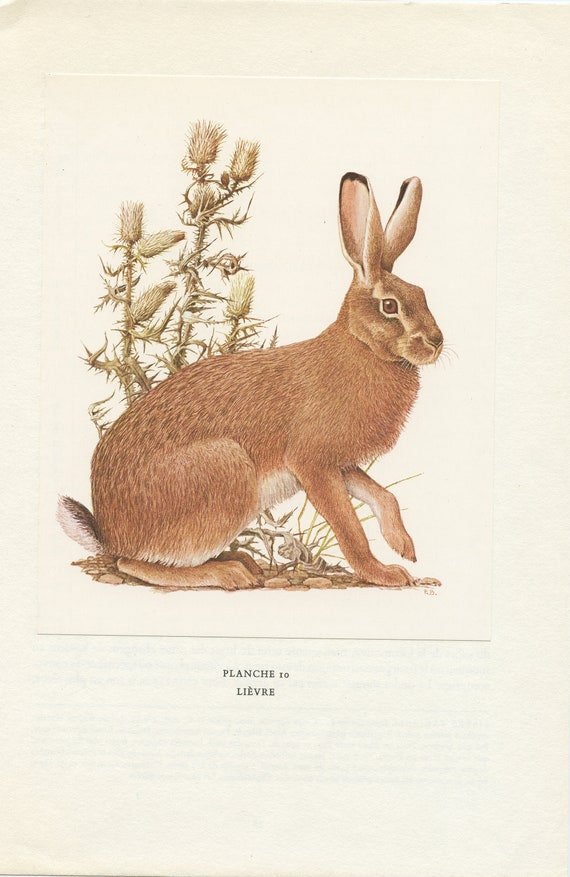This image features an intricately detailed, hand-drawn depiction of a brown bunny with black-tipped ears standing on a small patch of pebbled dirt. The bunny is centered prominently against an off-white, manila backdrop, reminiscent of an illustration from a historical or scientific book. One of the rabbit's forefeet is lifted, while the other three remain grounded, giving it a poised stance. The bunny's gaze, with one brown eye, is directed towards the viewer, creating an engaging focal point.

Behind the rabbit, there's a light green, prickly vine or foliage that adds a natural element to the scene. Additional foliage is visible between the rabbit's front and back hooves. The entire scene exudes a muted, yet naturalistic palette, enhancing the illustration's timeless quality.

The bottom third of the illustration is predominantly blank, except for a line of text beneath the bunny. The text, which appears to be in French, reads "Planche 10 Le Verre". This captioning supports the notion that the image is from a book, possibly a scientific or historical compendium.